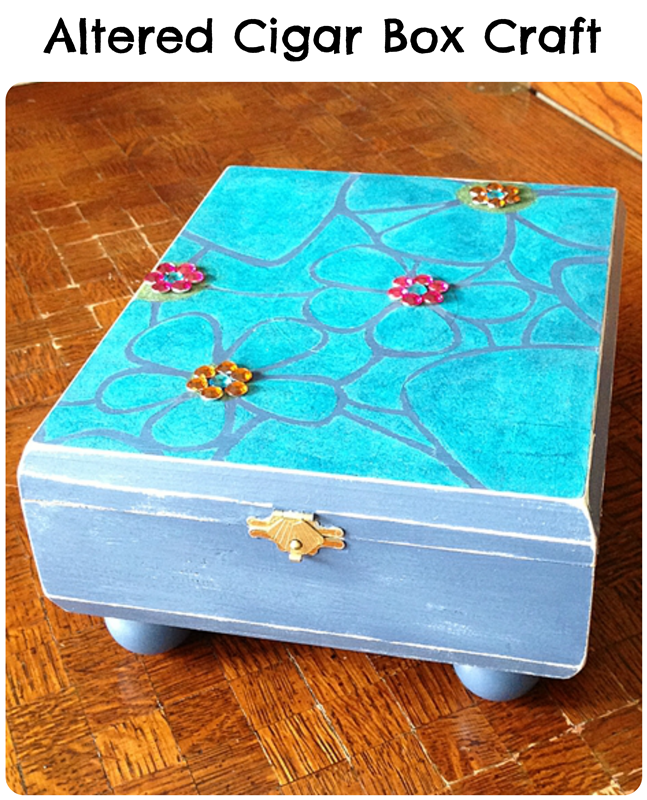The photograph depicts a child's craft project, labeled "Altered Cigar Box Craft," showcasing a skillfully upcycled cigar box. This decorative box features a striking paint job in varying shades of blue, with the main body painted a medium blue and the top a turquoise blue. The top surface is adorned with hand-drawn floral patterns in a slightly different blue and pale lilac. At the center of these floral drawings are crystals, two in gold or yellow and two in pink or purple. These flowers, which appear to be made of metal, are intricately designed with details reflecting abstract artistry. 

Adding a sense of elegance, a small golden clasp secures the front of the box. The box is also set on light blue feet, adding to its crafted charm. This decorative piece is placed on a slightly worn, brown, wooden parquet floor that exhibits a classic checkerboard pattern. The backdrop includes a wooden door and baseboard, providing a warm, earthy contrast to the box's cool tones. The image is topped with a caption in black typeface that reads "Altered Cigar Box Craft," highlighting the creative transformation of an everyday object into a delightful artistic piece.